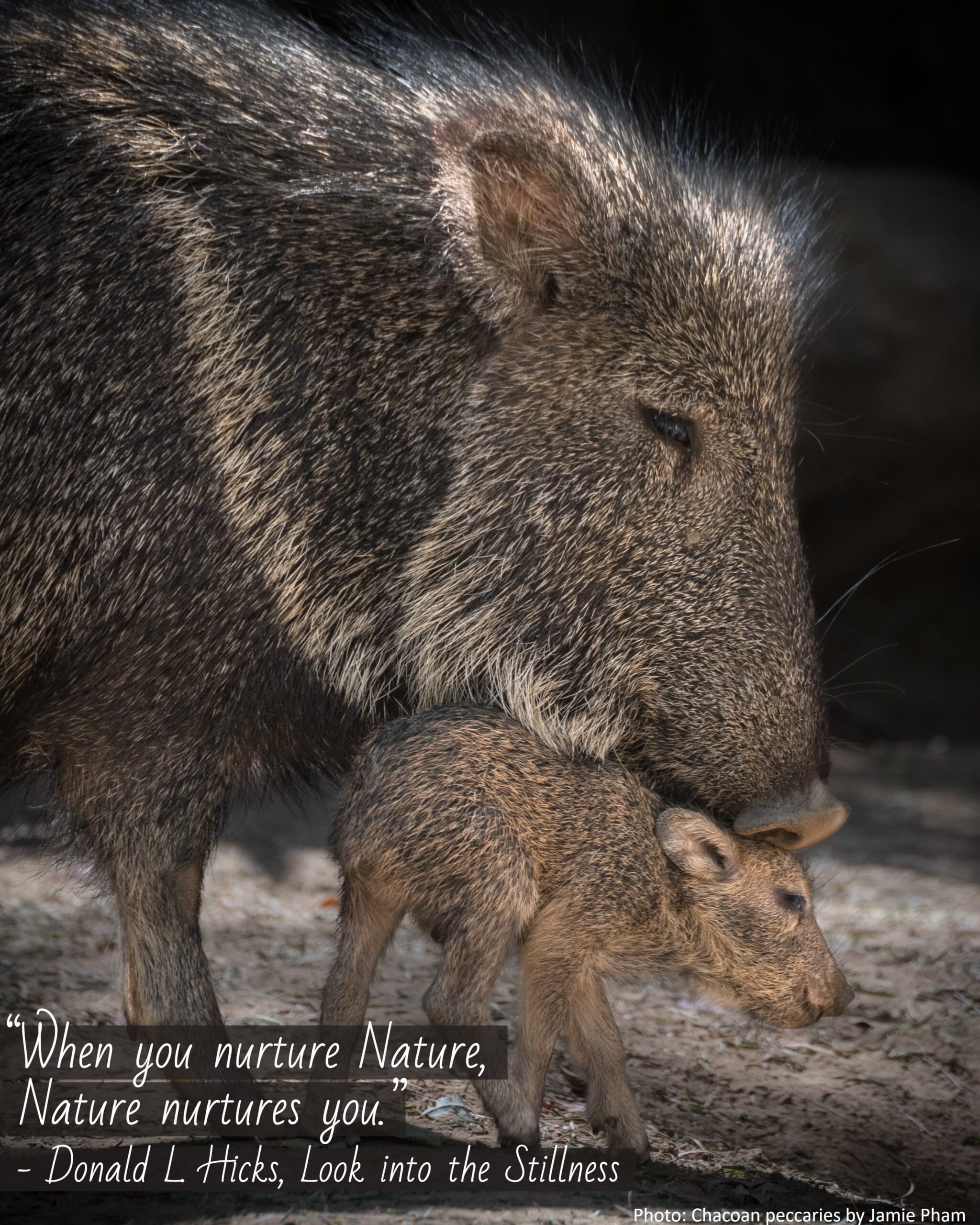This vibrant color photograph captures a tender moment between a mother javelina and her baby, both in profile. The mother, showing her dark brown and black fur interspersed with specks of white, is prominently featured from just behind her front legs. She enters the frame from the left and faces right, her head bent gently forward and resting atop her baby, creating a touching pose of protection and affection. The baby javelina, which sports a slightly lighter brown and black coat, stands beneath the comforting weight of its mother's head. Providing an evocative touch, the bottom of the image displays a poignant quote in white text: "When you nurture nature, nature nurtures you. Donald L. Hicks, look into the stillness."